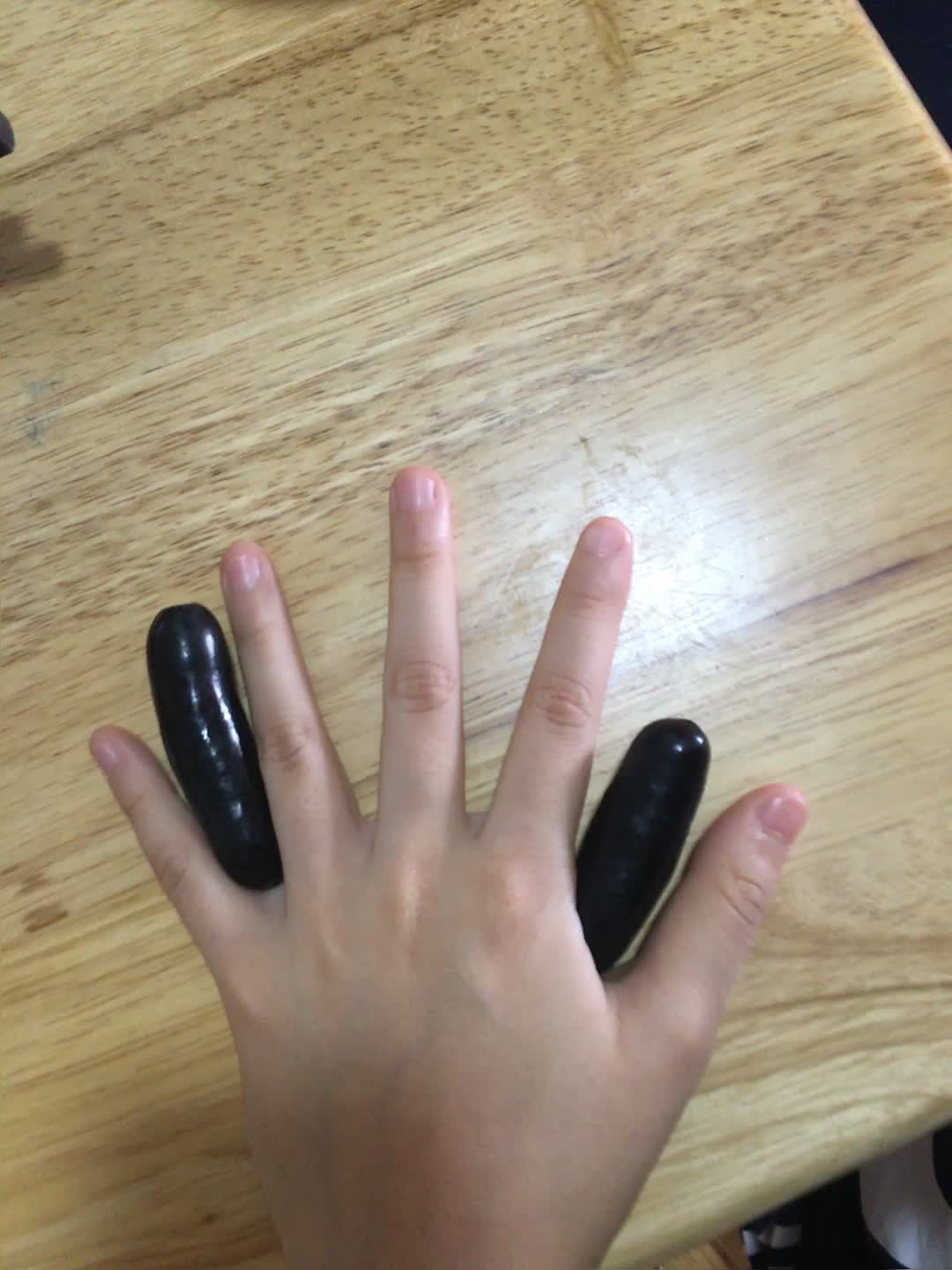A top-down photograph captures a light-skinned person's left hand laying flat on a light brown, wooden table with darker speckles. The fingers are evenly spread apart, showing short, slightly flushed pink fingernails. Two shiny, cylindrical, black objects resembling cucumbers or possibly pickles or jalapeno peppers are positioned between the fingers. One object is nestled between the pinky and ring fingers, and the other is between the thumb and index finger. The black objects vary slightly in glossiness and shape, with the one between the pinky and ring fingers appearing longer and glossier, while the one between the thumb and index finger is of similar length to the thumb. The table’s edges are visible in the lower and upper right corners, adding context to the placement of the hand and objects.